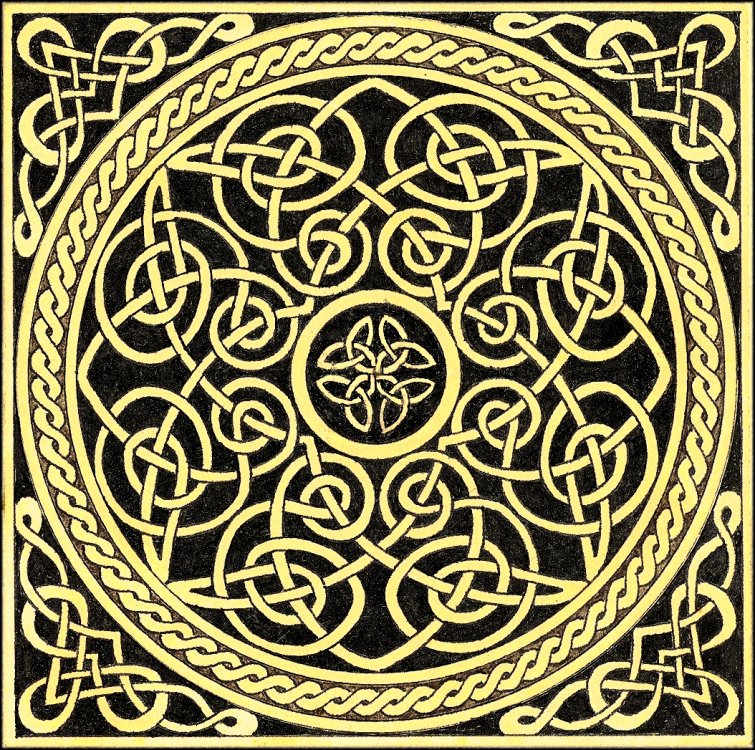The image showcases an intricate and ornate design known as polyhedra in knots. Set against a black background, the artwork is dominated by an off-yellow color, creating a striking contrast. Each of the four corners features identical, interwoven Celtic knot designs, incorporating intricate swirls and triangles. Moving inward, a large rope-like or braided circular pattern encircles the central area. Within this circle, another concentric ring contains a detailed, criss-crossing knot design. The central motif also features additional loops and interlocking patterns, forming an elaborate and symmetrical composition that could embellish anything from a quilt square to a stained glass piece. The overall design conveys a sense of unity and repetition, with each ornate section and corner intricate yet cohesive within the larger framework.